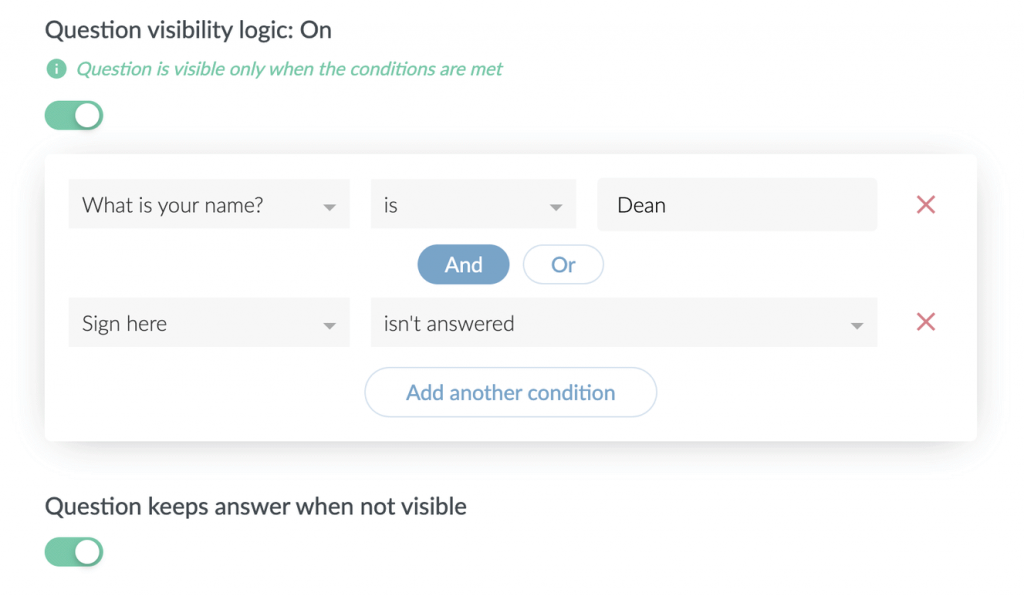The image depicts a user interface for configuring conditional visibility settings in a form setup. At the top, there is a section labeled "Visibility Logic: ON," highlighted in green text with a green circle containing an eye icon. This section indicates that the visibility of a question is dependent on certain conditions being met.

Below, a green-filled slider bar further reinforces the "ON" status for visibility logic. Underneath the slider bar, there are multiple text boxes and dropdown menus. The first dropdown menu is labeled "What is your name?", followed by an adjacent text box pre-filled with the name "Dean" and marked with a red X, suggesting an error or invalid entry. Next to this is a blue button labeled "AND" and a white button labeled "OR."

Further down, another dropdown menu appears with a similar invalid entry indicated by a red X. To the right of this menu, there is a white button with blue text that reads "Add Another Condition," allowing the user to include additional criteria.

At the bottom, there is another section titled "Question Keeps Answer When Not Visible," accompanied by a green-filled slider bar, indicating that this feature is active.

The entire interface is set against a clean white background, emphasizing clarity and usability.